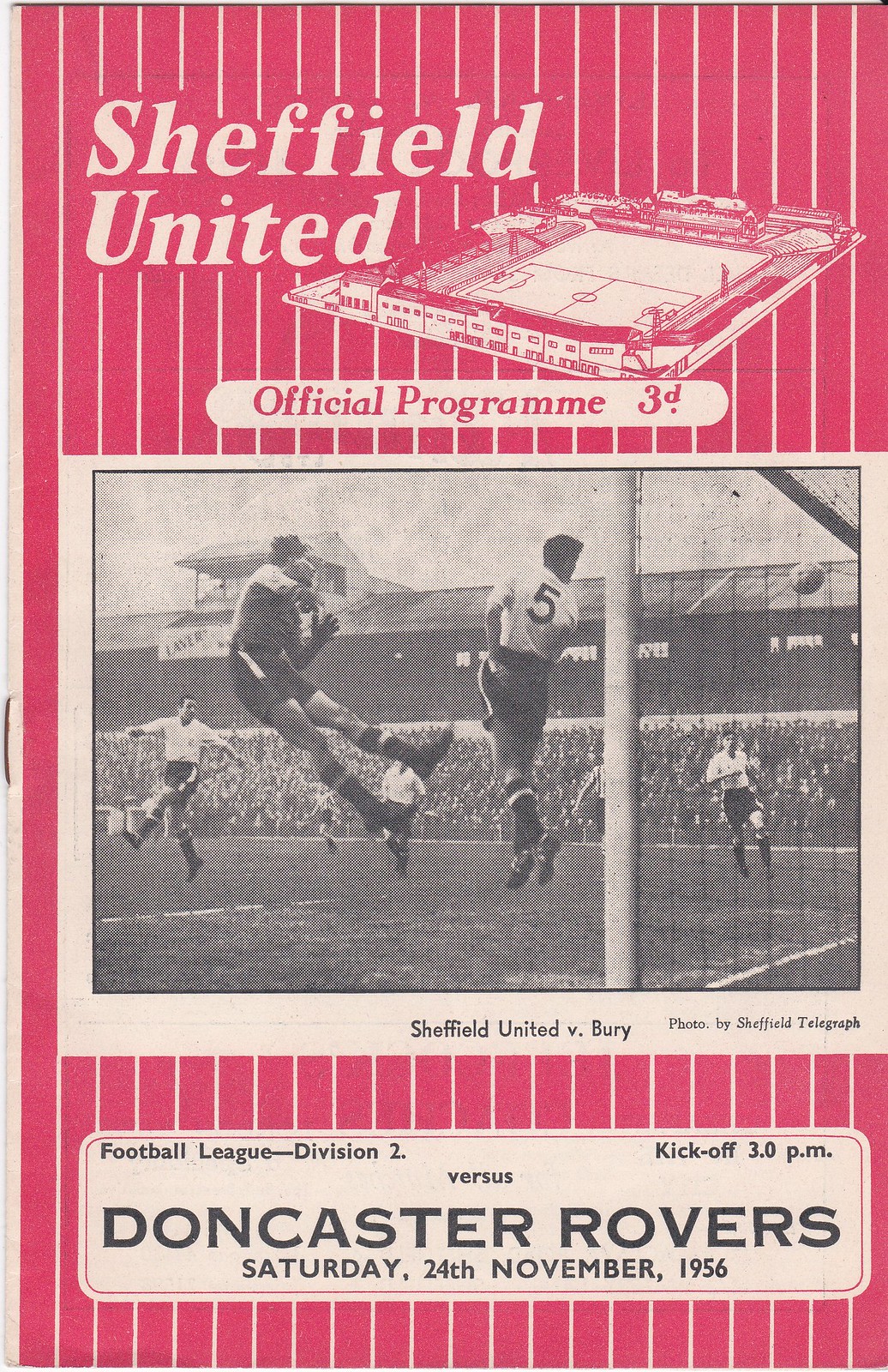This is a color photograph of the front cover of the Sheffield United football team's official program. The background is predominantly light red with white pinstripes. Dominating the center is a black-and-white photograph taken outdoors on the soccer field, capturing an action-packed moment of a game. In the foreground, two soccer players are captured mid-air in a leap, while several other players can be seen running or jumping in the background. The text on the cover reads "Sheffield United versus Bury (B-U-R-Y), Football League Division 2, Kickoff 3 p.m." Additionally, it mentions "Sheffield United versus Doncaster Rovers, Saturday, 24th November 1956." The photograph is credited to Sheffield Telegraph. The cover also includes the price, noted as "3D."